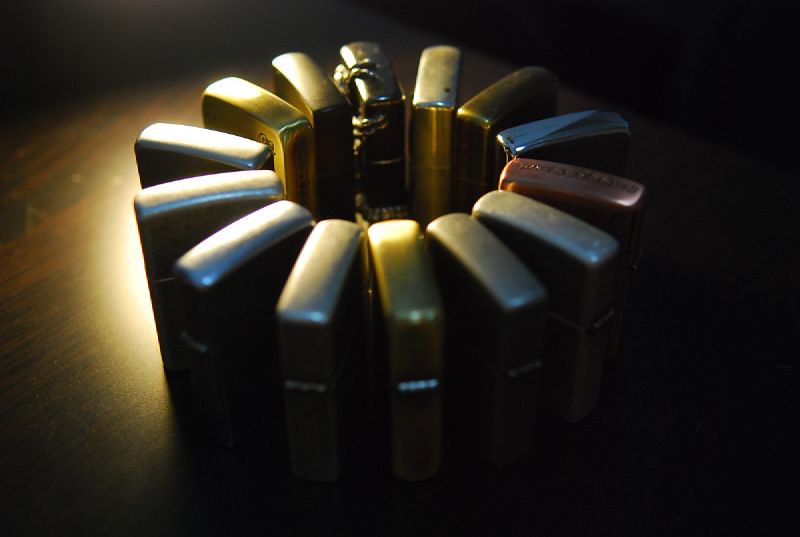In an atmospheric indoor photograph featuring a dark, blacked-out background with minimal lighting, a collection of Zippo brand cigarette lighters is meticulously arranged in a circular formation on a wooden tabletop. The dim light source emanates from above, creating a soft white shadow on the middle-right of the table and subtly illuminating the surface. This careful arrangement consists of 14 lighters, predominantly silver, gold, and bronze. The detailed lineup includes variations: a black and silver lighter, a gold lighter, gold and black lighters, copper-colored ones, several brushed gray and worn silver ones, and a notable lighter at the top of the circle with intricate rope-like detailing. Among these, one lighter on the right side has a pinkish or maroon hue, adding a unique splash of color to the composition. The image's slight out-of-focus quality lends an artistic blur, while the contrast between the dark background and the metallic sheen of the lighters captures the viewer's attention, making the scene thoughtfully dramatic.